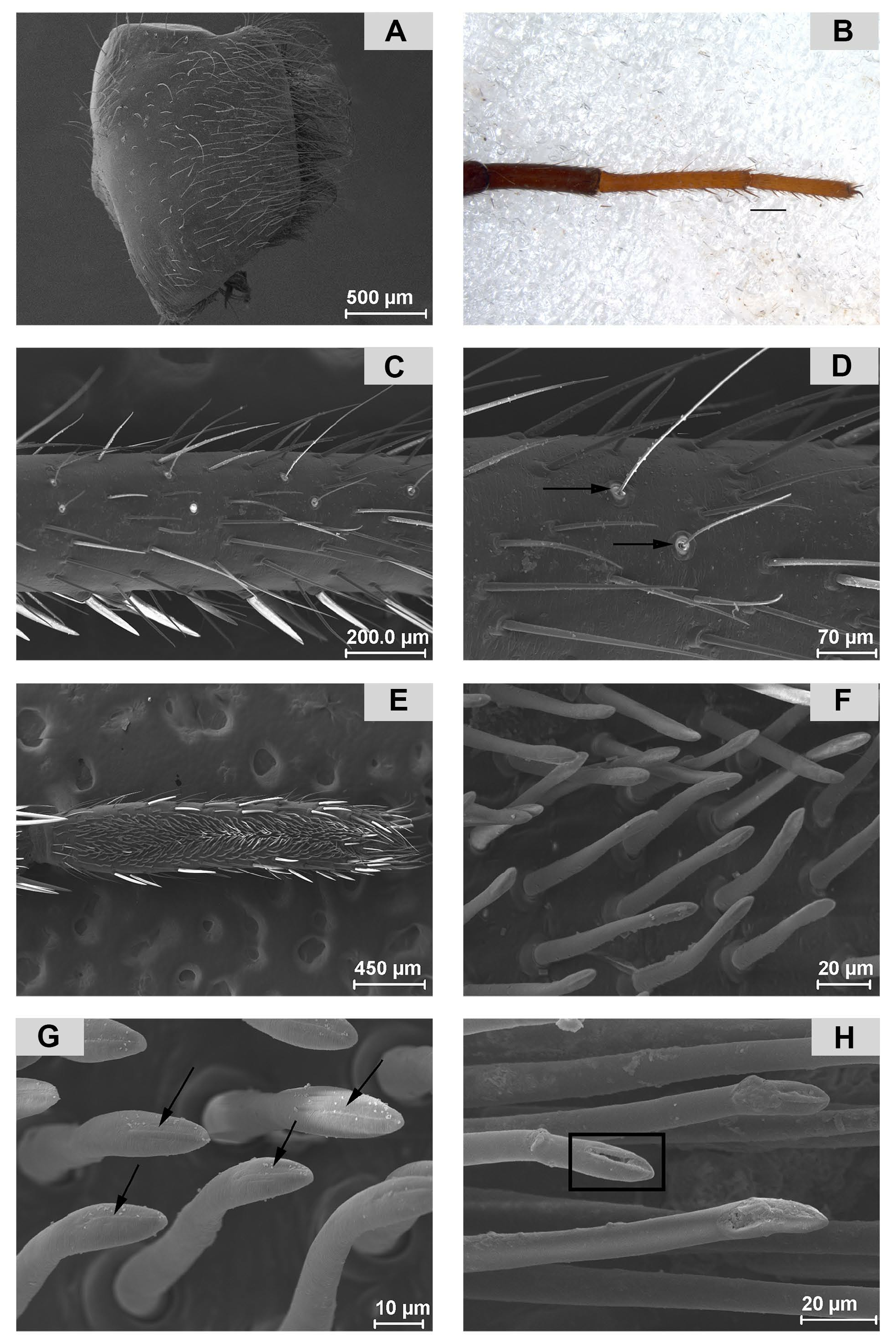The collage presents a series of eight detailed microscopic images labeled from A to H, capturing various magnified views of an insect leg. Image A, the only one with color, showcases a heart-like structure with fine strings extending from it, and a 500 micrometers scale bar is visible on the bottom right. Images B through H are in black and white, progressively zooming in on specific parts of the insect leg. Image B features a single, dark to light brown bug leg segment against a white background. Images C and D provide a closer look at the leg's intricate structures, with magnification scales of 200 and 70 micrometers respectively. Image E zooms further to focus on one particular hair, showing fine details at 450 micrometers. Image F reveals numerous tiny hairs on the leg, captured at a scale of 20 micrometers. Image G, with annotations pointing at the hairs, offers a more intensified view at 10 micrometers. Finally, image H, at 20 micrometers, zooms out slightly, providing a broader view of the leg's hair structures. Each image is meticulously labeled with scales denoting micrometers, showcasing the high-magnification detail achieved by the powerful microscope.